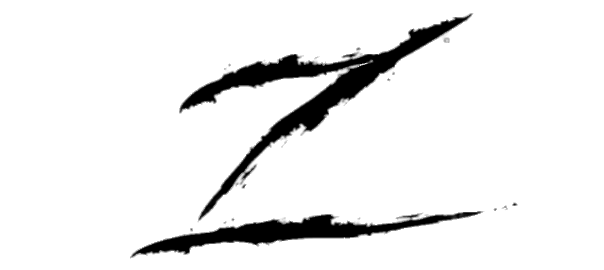A bold, black "Z" logo, inspired by the iconic "Z" of the Zorro character, dominates the scene. The design features jagged lines, giving it a rugged and dynamic appearance. The top segment of the "Z" is a short yet bold horizontal stroke. The central part slashes diagonally from the upper left to the lower right, intersecting the entire symbol. Completing the character, the bottom segment forms another horizontal stroke, mirroring the top line but slightly disjointed. Adding a touch of contrast, faint white edging outlines the entire "Z," giving it a subtle, almost ethereal highlight against the darker backdrop.